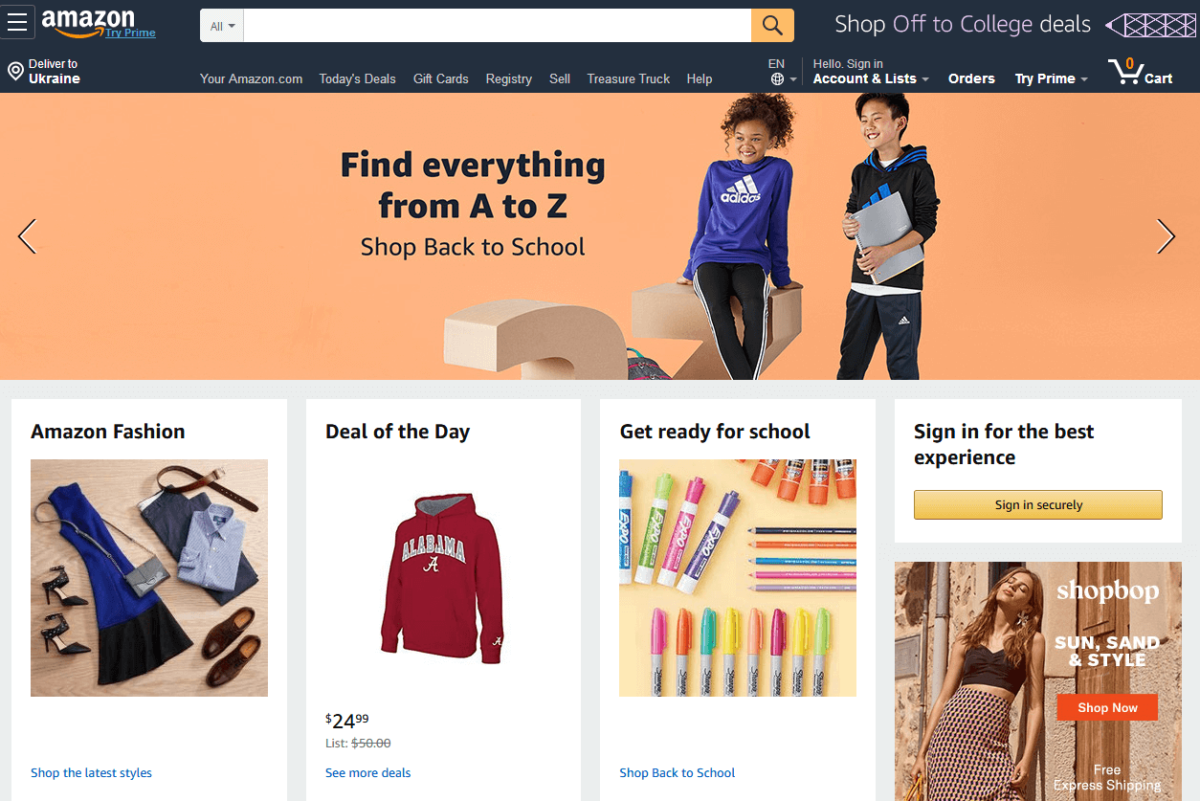The image depicts a detailed screenshot of the Amazon website homepage. The top section features a black banner, where on the left side there are three horizontal white lines stacked vertically within a square, representing the menu icon. Next to the icon, "Amazon" is displayed in white text with an orange arrow beneath it. To the right, "Tri-Prime" is written in blue lettering with an underline, indicating a special service or promotion. Below this, the text "Deliver to Ukraine" appears, with "Ukraine" in bold print and capitalized.

Continuing across the top, there is a search bar labeled "All" with a drop-down arrow, followed by an orange square with a magnifying glass icon inside. To the right of the search bar, a promotional banner reads "Shop Off to College Deals," illustrated with a purple or purplish-pink pencil drawing.

Below the banner, several navigation links are present: "Your Amazon.com," "Today's Deals," "Gift Cards," "Registry," "Sell," "Treasure Truck," and "Help." Additionally, language options, as indicated by "English," and account-related links such as "Hello, Sign In," "Account and Lists," "Orders," and a "Tri-Prime" link are displayed. At the rightmost end is a shopping cart icon with a count of "0" highlighted in orange.

The background features a peachy-orange promotional section stating "Find Everything from A to Z, Shop Back to School" with "Find Everything from A to Z" in bold print and the letters "A" and "Z" capitalized. This section also includes a graphic of two children dressed in athleisure wear.

The bottom part of the image highlights promotional tags such as "Amazon Fashion," "Deal of the Day," "Get Ready for School," and an invitation to "Sign In for the Best Experience."